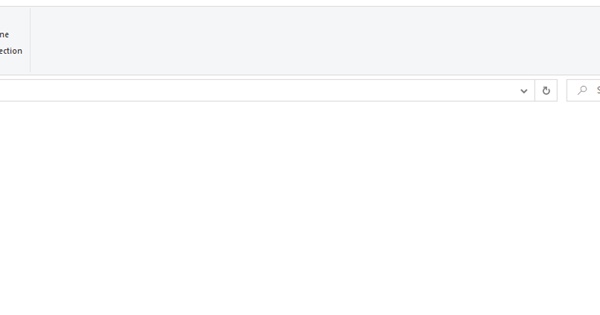The image depicts the top section of a digital web interface. The upper part of the screen is shaded in a light gray color, extending horizontally from the left edge to the right edge of the image. A faint vertical gray line intersects this area. In the upper left corner, partial text is visible, specifically the letters "N" and "E" in black print. Below this, the sequence "E-C-T-I-O-N" appears, suggesting the word "SECTION," with a vertical line separating this text from the adjacent area.

Further down, a drop-down menu is indicated by a downward-pointing arrow located in the far right corner of the screen, though the contents of the menu are not visible. To the right of this drop-down menu area, there is a refresh button and a magnifying glass icon, typically used for search functions, situated towards the right side of the image.